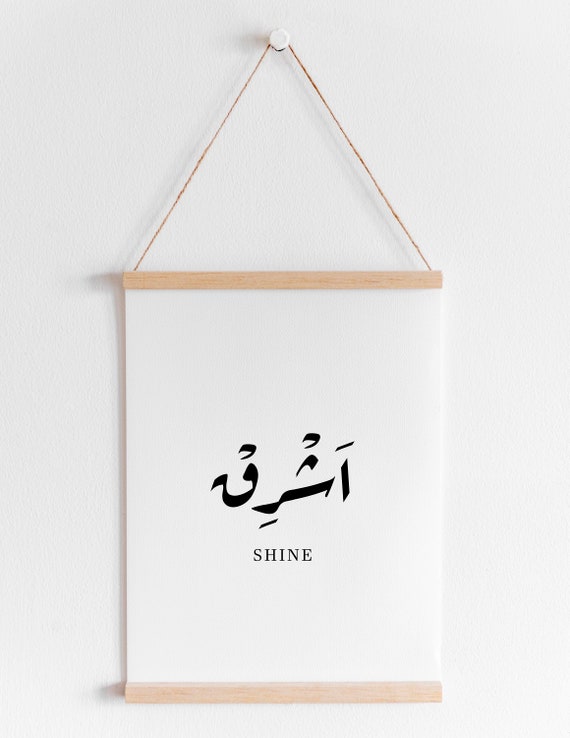The photograph depicts an indoor scene illuminated by artificial light, featuring a vertically rectangular composition with a gray wall as the background. The lower right corner of the image is notably faded, suggesting it is hit by a light source. At the top center of the image, a white thumbtack is embedded in the wall, from which a tan or brown string is suspended, forming a triangular shape. Hanging from this string is a piece of white parchment or paper, bordered by light tan or brown wooden strips at the top and bottom. The paper features an inscription in black, possibly Arabic, consisting of three characters that might resemble musical notes. Below this inscription is the English word "SHINE" written in all capital letters.